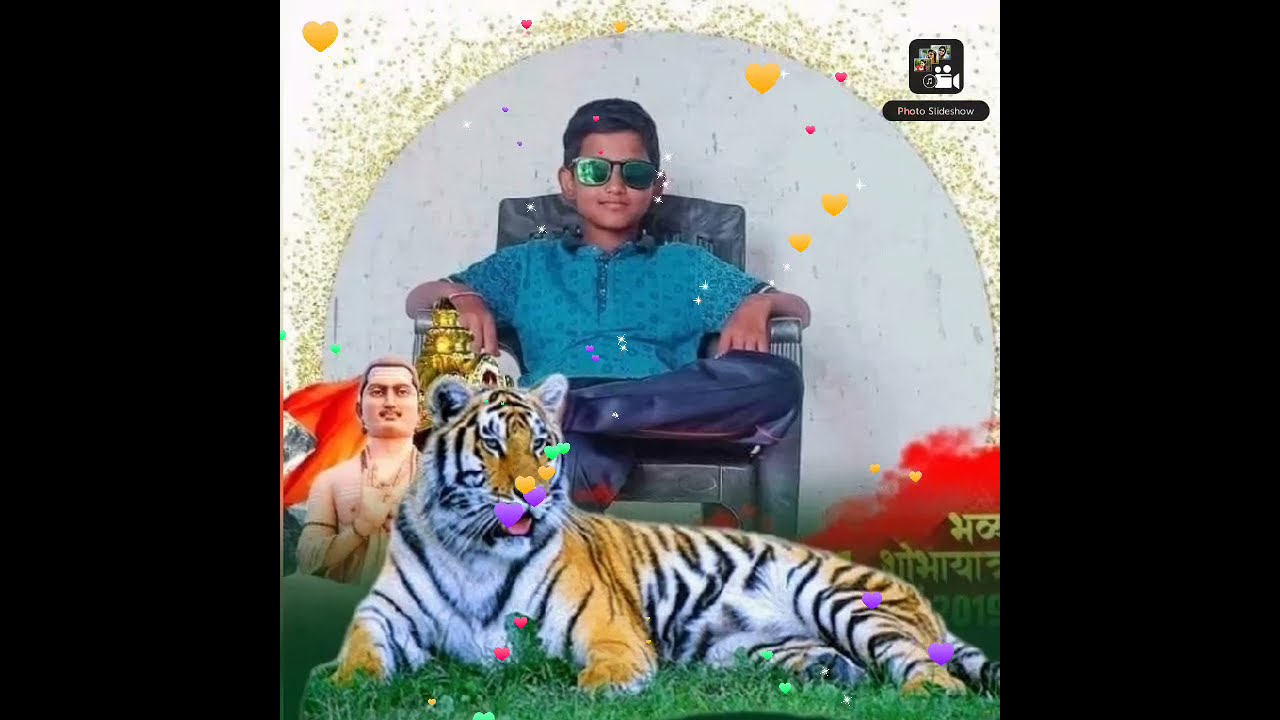This is a detailed and edited photograph of a young boy, approximately 10 to 12 years old, sitting on a green chair with a crossed leg posture, where his left leg is over his right. The boy, with short black hair and slightly darker brown skin, sports green-lensed sunglasses, a short sleeve blue patterned button-down shirt, and black or gray slacks. The background features a cream-colored base adorned with dotted patterns behind a white semicircle. Below him, an edited image showcases a white tiger with orange and black stripes lying on green grass sprinkled with pink and green flowers. Near the tiger, there is an edited statue of a man, portrayed shirtless with brown hair and his right hand on his chest, accompanied by an orange flag behind it. Various colored hearts—orange, pink, green, yellow, and purple—are scattered throughout the image as a filter. Additionally, the top-right corner of the picture includes a logo with the text "Photo Slideshow," and the image is flanked by two black vertical strips on both sides, forming a solid border.